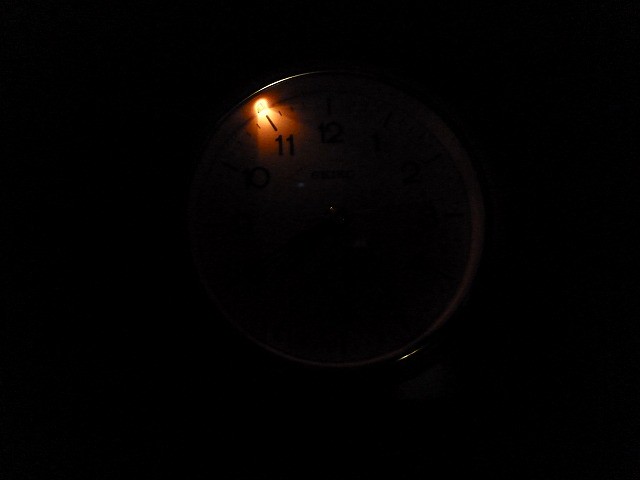The image is predominantly black, with a dark background that extends across the entire frame. At the center, there is a circular object resembling a clock or stopwatch. This circular figure has small dashes between the numbers, and longer dashes where the numbers are located. The numerals 10, 11, and 12 are visible at the top left portion of the object, with a bright, possibly yellowish light illuminating the 11. The material of the clock or stopwatch gives the highlighted area around 11 a coppery, brownish appearance. There is a faint reflection of light on the bottom right edge, subtly outlining the object's circular form. Overall, the image is very dark, with only these details discernible.